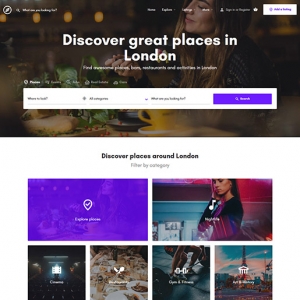The image showcases two distinct sections of a web page dedicated to London. The upper section features a rectangular banner with a dark overlay. The background of this banner appears to be a woman, possibly in a restaurant, reaching for something on the table. Despite the dark overlay, her face and right hand, along with some greenery and table elements, are slightly visible. Overlaid on this background in white font is the slogan "Discover Great Places in London," accompanied by a centrally placed search bar below the text.

The lower section, seamlessly flowing from the upper banner into a single web page with a white background, contains the instructional text "Discover places around London. Filter by category." Beneath this text, there are two wide rectangular images side by side, each with two smaller square images below them, maintaining the same total width. These images display various elements related to different categories and are accompanied by relevant icons, such as a person playing a musical instrument with a musical note symbol and a picture of dumbbells paired with a dumbbell logo. This layout and design effectively categorize and visually guide users in their exploration of London's offerings.